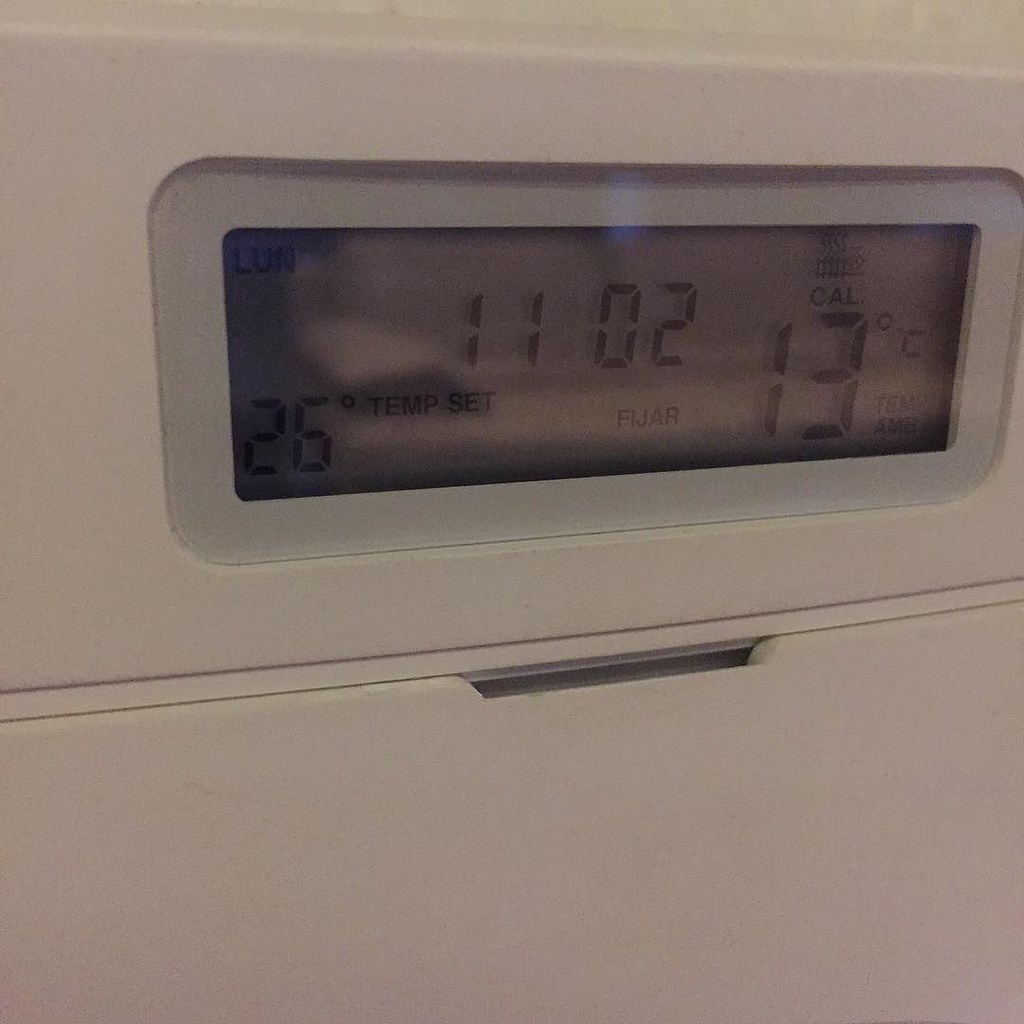Image Caption: 

The photograph depicts a thermostat against a stark white background. The thermostat, mounted securely on a white wall, features a prominent digital display screen set within a rectangular, grayish-blue plastic bezel. The display screen shows various readings and is divided into different sections. In the upper left corner, the word “low” is visible, while in the lower left corner, the text reads “26 degrees temp set.” Centrally displayed is the time, “1102,” below which the term “FIJAR” is displayed. To the right of this, the screen indicates “CAL 13 degrees Celsius.” Beneath the display screen, there are two horizontal lines extending from left to right, and a noticeable rectangular black piece missing from the bottom, resembling a detachable drawer or access panel.